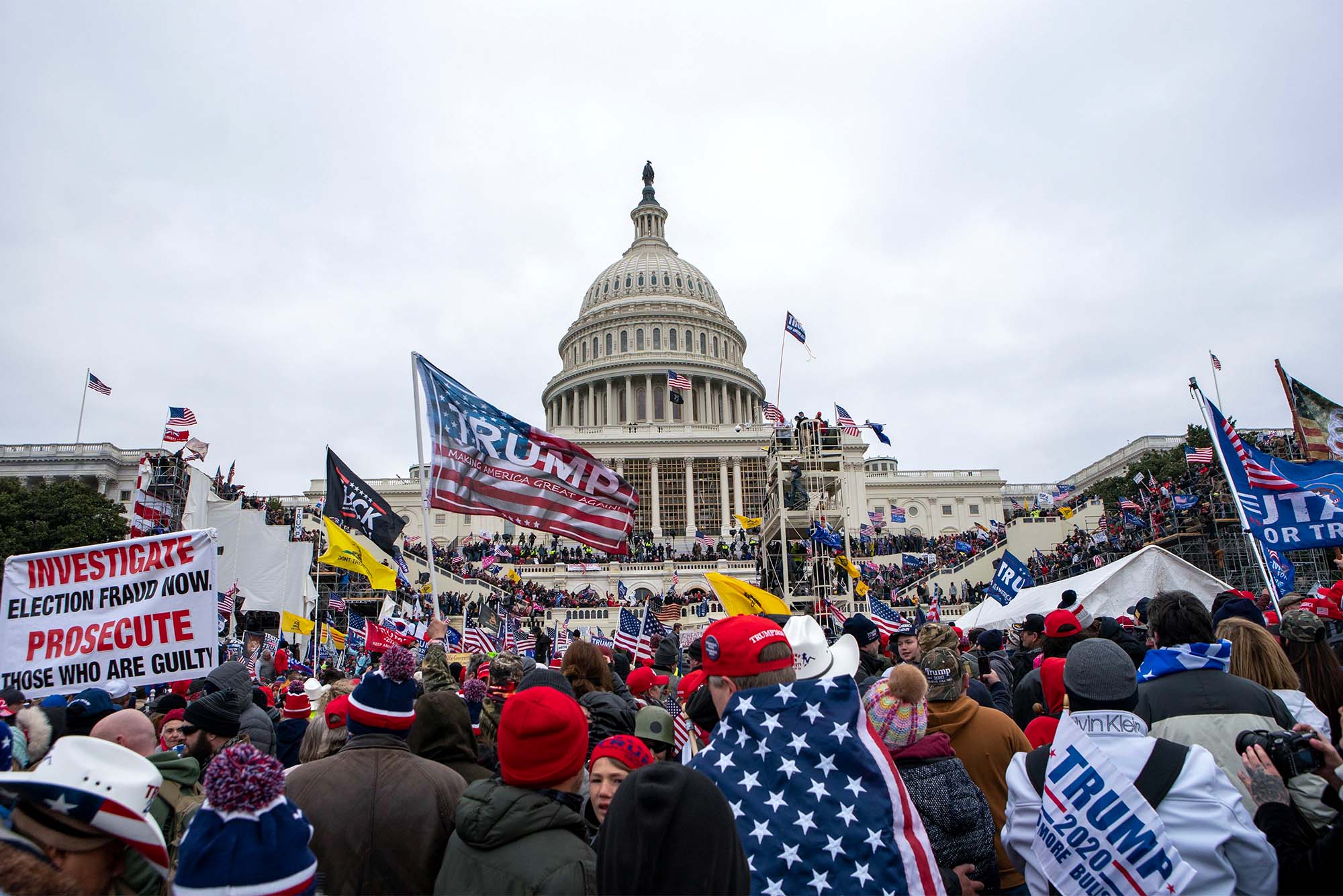The photograph captures the chaotic scene in front of the U.S. Capitol building during the January 6th rally, with an overwhelming crowd of Trump supporters enveloping the area. The image, taken on a gray winter day, beautifully frames the Capitol at the center, its iconic dome standing tall against the cloudy sky. The tightly packed crowd, donned in warm clothing, red and blue hats, and adorned with American-themed outfits, showcases a profusion of flags and signs. Predominant among the flags are those bearing "Trump 2020" and classic American designs, interspersed with five "Don't Tread on Me" yellow banners. Multiple signs proclaim "Investigate election fraud now, prosecute those who are guilty," reflecting the rally's fervent agenda. The image underscores both the size and the intensity of the assembled mass, all fixated on the Capitol, providing a stark portrayal of that significant and contentious day.